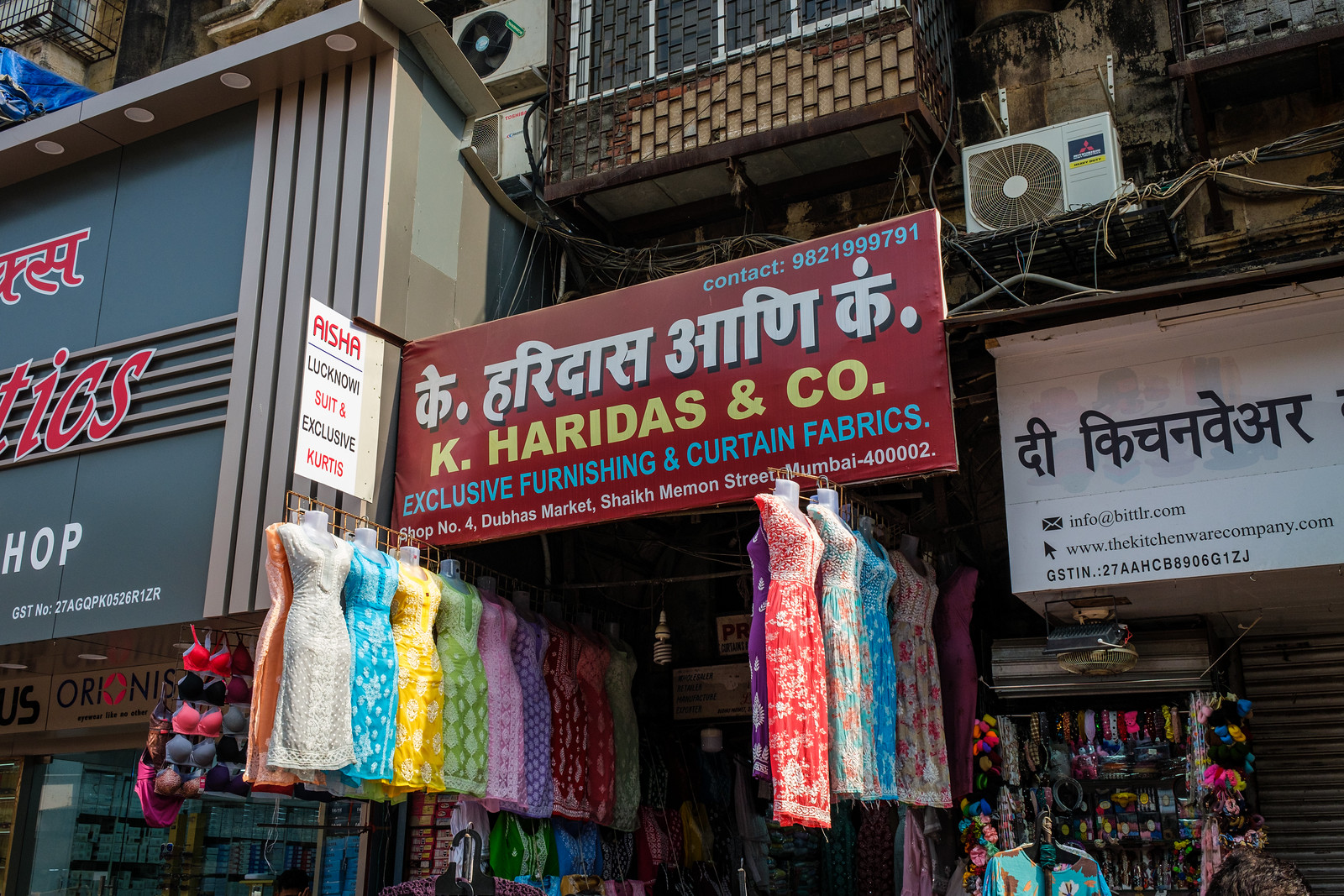In this vibrant street scene, a bustling neighborhood is captured with a mix of commercial and residential structures. The focus is a shop at the center of the image, prominently displaying a dark red sign with both Hindi writing and the words, "K. Haridas & Co. Exclusive Furnishing and Curtain Fabrics." The shop showcases an array of vibrantly colored dresses, displayed on armless and headless mannequins at the entrance. These dresses feature various hues, including gray, light gray, blue, yellow, green, light lavender, purple, red, and more. Adjacent to the dresses, a variety of brassieres in colors ranging from red to black are also hung out for display. Flanking this main store, other shops with storefronts in gray and red, feature signage in Hindi. A gray storefront on the far left has partially visible red letters spelling "TICS" and "shop" in white below. The upper floor of the buildings shows residential apartments with numerous window air conditioning units visible, adding to the urban, lived-in feel of the neighborhood.